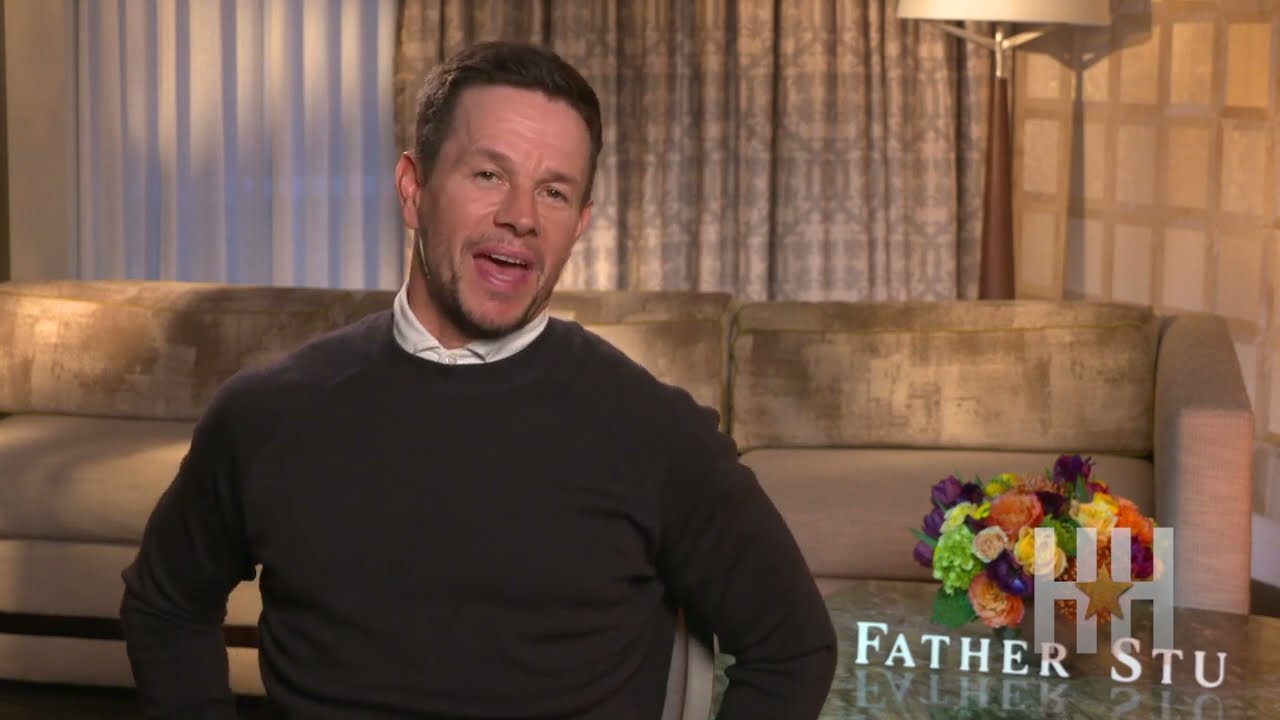In the image, we see Mark Wahlberg sitting in what appears to be a staged living room setting, likely intended to resemble a grandmother's home, possibly for a promotional or press interview. Mark is positioned directly in the center, looking straight at the camera with his mouth slightly open. He is dressed in a dark grayish-brown sweater vest layered over a white button-down shirt. He has a clean haircut, a light beard, and short brown hair.

Behind Mark is a long beige couch, partially obscured by cream-colored curtains with a beige pattern, which suggest a cozy indoor environment. To the right, there is imitation paneled wallpaper and a brown lamp. In the bottom right corner of the image, there is a table with a colorful bouquet of flowers on it. Overlaid on the image in the bottom right corner is the text "Father Stew," which appears graphically edited to look like it's reflecting off the table surface. Above this, the letters "HH" with a star in between are also reflected similarly, contributing to the promotional aspect of the setup. The predominant colors in the image are light brown, beige, white, pink, purple, green, orange, yellow, and red, which come together to create a warm and nostalgic atmosphere.